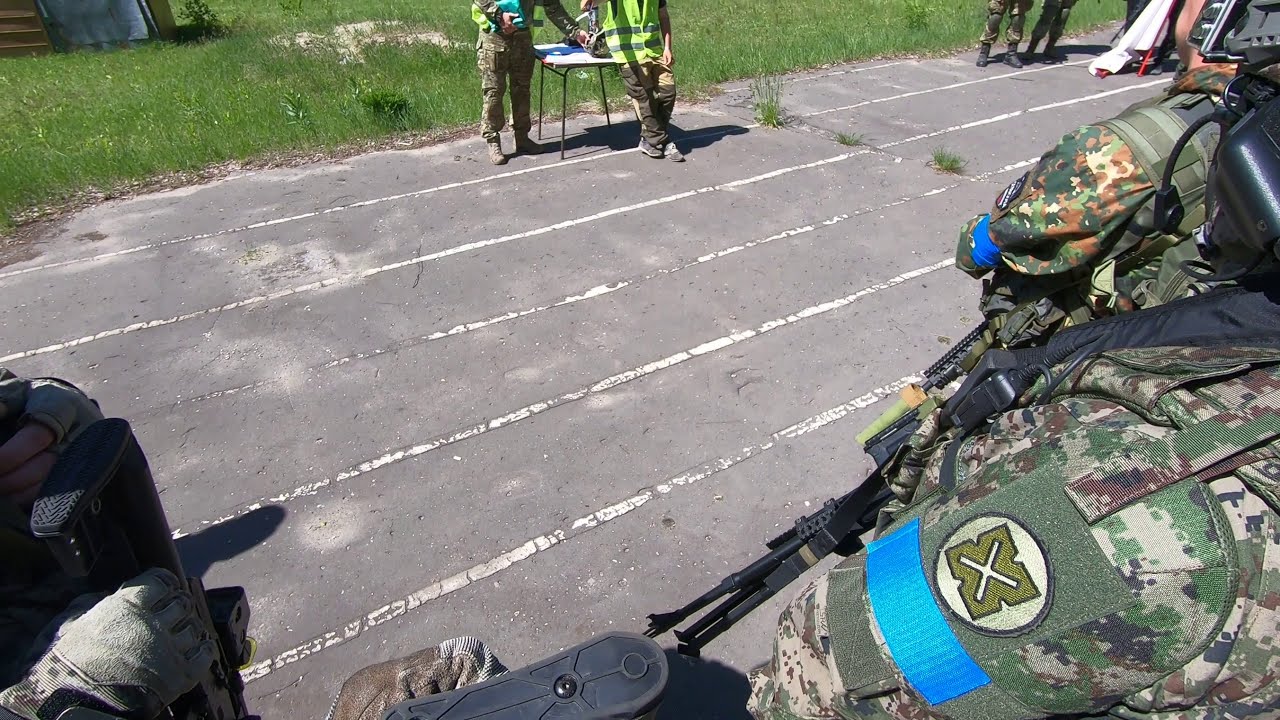In the image, taken during the daytime with sunlight, an asphalt road marked with five straight white lines spans the middle. At the top center, two individuals in military uniforms, with a green digital camouflage pattern, wear fluorescent safety vests and stand in front of a small table. The scene is further detailed with lush green grass on the side, indicating an outdoor environment. In the bottom right corner, the shoulder of another person in uniform is visible, featuring an insignia of a green X cross with a blue line below it. The individuals, possibly soldiers or military personnel, are equipped with various gear, including boots, and appear to be participating in some type of training or instructional activity. Additionally, there is a small shed or structure visible in the background. The perspective of the image suggests it might have been captured from a body cam.